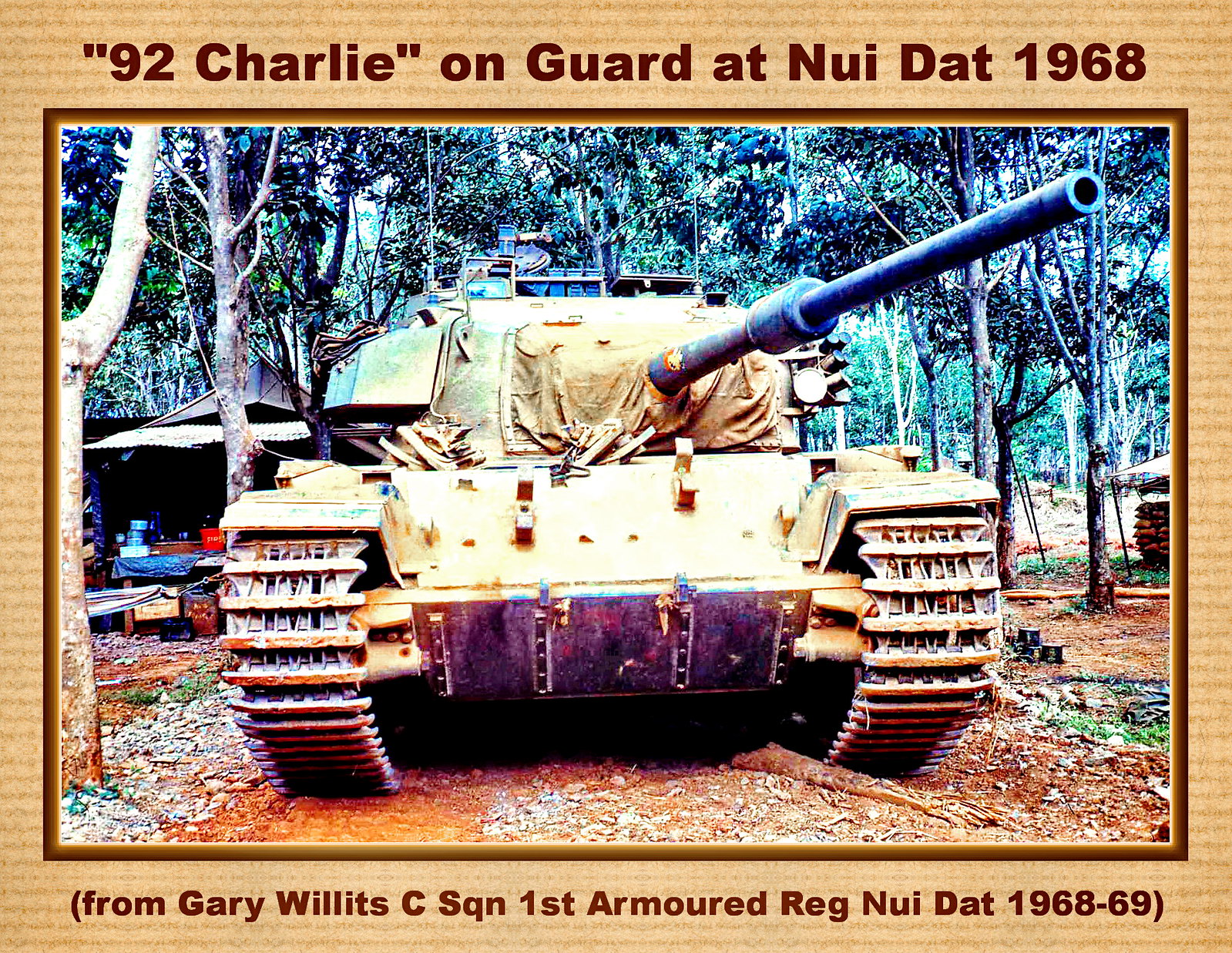The photograph in the center of the image captures a large U.S. Army tank, painted in a brownish hue, with a prominently protruding cannon. The tank is parked on a dirt patch, surrounded by a densely forested area suggestive of a campsite in Vietnam. To the right of the tank, a wooden structure is partly visible, while to the left, there appears a tent or shack-like building accompanied by tables under an awning, laden with cans and a blue tarp. Behind these elements, numerous trees contribute to the background scenery. Notably, the image lacks any visible personnel. Encapsulated within a brown and tan striped border, the photo is identified by text at the top which reads, "92 Charlie on guard at Nui Dat, 1968," and is further credited at the bottom, "From Gary Willits, C Squadron, 1st Armored Reg, Nui Dat, 1968-1969."